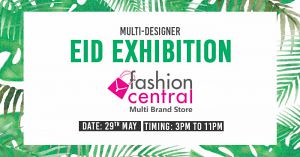The promotional flyer for the store event features a vibrant border composed of various tropical plant leaves, including ferns and palm tree leaves. At the center of the flyer, a white rectangle serves as the backdrop for multiple lines of text. 

From the top, in black text, it reads "multi-designer," followed by green text announcing an "EID exhibition." Further down, "fashion" is displayed in black text with the loop of a 2D purse creatively wrapped around the 'F'. Underneath "fashion," pink text spells out "central," and at the bottom of this section, black text reads "multi-brand store."

Towards the bottom of the image, there are two black rectangles: the left one contains white text that details the date, "29th May," and the right one lists the event timing, "3pm to 11pm," also in white text. The flyer is small and rectangular, resembling a business card, with the longer side on the x-axis.